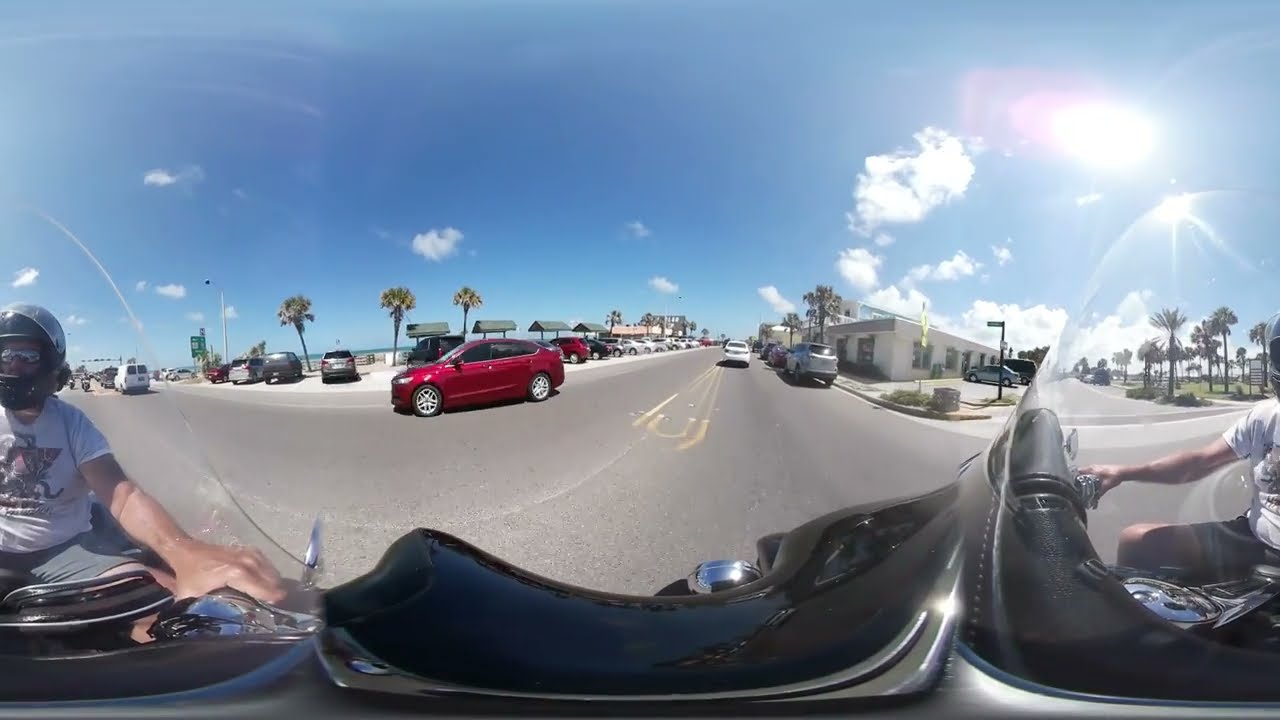This panoramic 360-degree image captures a beachside road scene as viewed from the front of a motorcycle. The image, which appears slightly distorted due to its immersive nature, showcases a motorcyclist in a white t-shirt and helmet, visible twice due to the wrap-around effect. Both sides of the road are visible, lined with tropical palm trees and a parking lot on one side. Various vehicles, including a silver sedan and a black pickup truck, can be seen driving on the road. The bright, sunny day is complemented by a blue sky with scattered puffy clouds, and a small strip of blue water is visible in the background, suggesting a seaside location. Additional elements like white and yellow road markings, a traffic light in the distance, and some parked cars near a green grassy area with a sidewalk add to the detailed landscape. In the center of the image, white text reads "Flagler Beach," reinforcing the beachside setting.